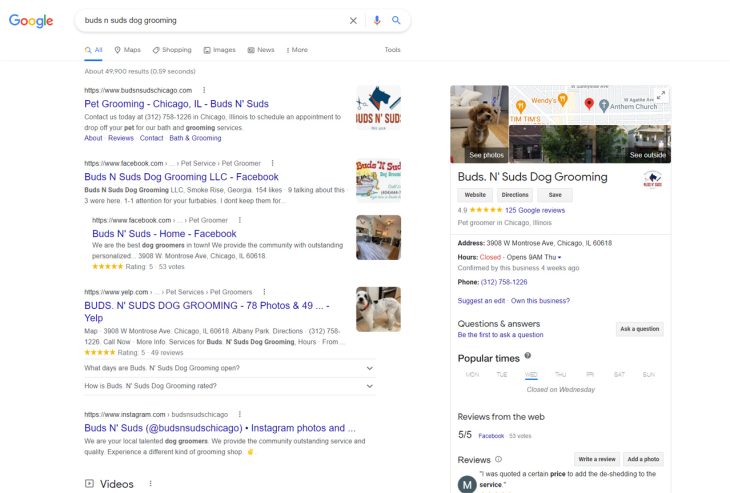This image is a detailed screenshot of a Google search page. In the upper left corner, the familiar Google logo is displayed in its traditional multicolored font. Centered prominently on the page is a search bar, within which the phrase "Buds and Suds dog grooming" is typed out. To the right of the search bar, the Google microphone icon and magnifying glass symbol are visible, signifying voice search and the search function.

The first search result is a clickable link to the website "www.budsandsudschicago.com". Below this URL, the text "Pet grooming, Chicago, Illinois, Buds and Suds" appears in blue. To the right of this text is a small square image containing the Buds and Suds logo.

Further to the right, there is a rectangular, gray-lined white box featuring a photograph of a brown and white poodle sitting on a rug in a comfortably furnished room with a couch. 

Adjacent to this photo is a small map illustration, pinpointing the location of Buds and Suds dog grooming. The map displays a red location pin near landmarks such as a Wendy's on the left and an Anthem Church on the right. Beneath the map, the caption reads "Buds and Suds dog grooming."